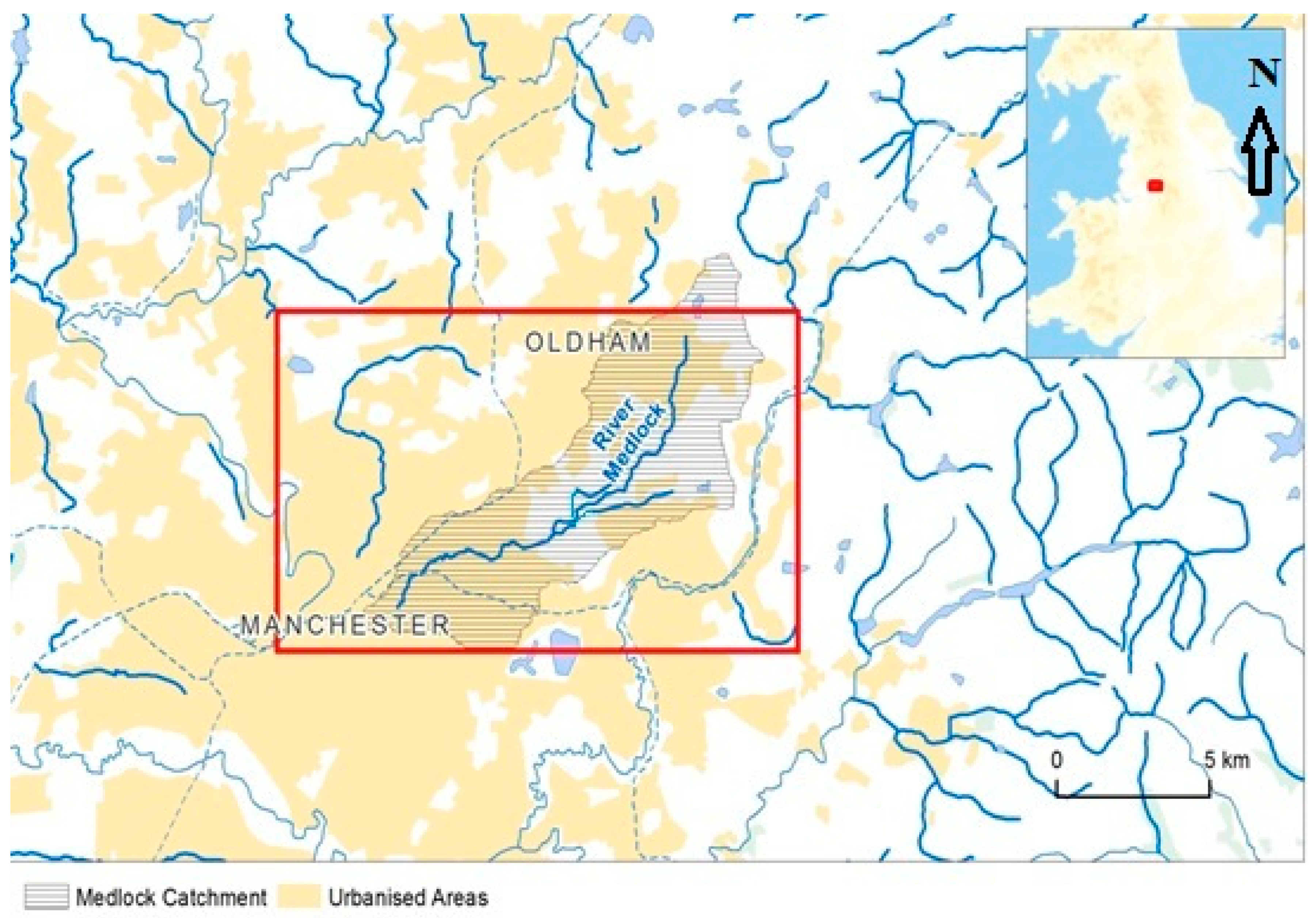This image is a detailed, bird's-eye view map of part of England, specifically focusing on the area encompassing Oldham and Manchester. The map features a red rectangle in the center, highlighting the Medlock Catchment area, which is delineated with gray stripes and includes the River Medlock flowing through it. Urbanized areas within the map are marked in yellow, indicating a high density of developed regions. Additionally, a smaller, zoomed-out map in the top right corner provides a broader view of the UK with a red dot pinpointing the specific area covered by the main map, showing the geographical context. The map includes a key in the bottom right corner to reference a distance of five kilometers, enhancing its utility for spatial understanding. An important feature in the top corner is a north arrow for orientation, ensuring the map reader can accurately interpret directions.